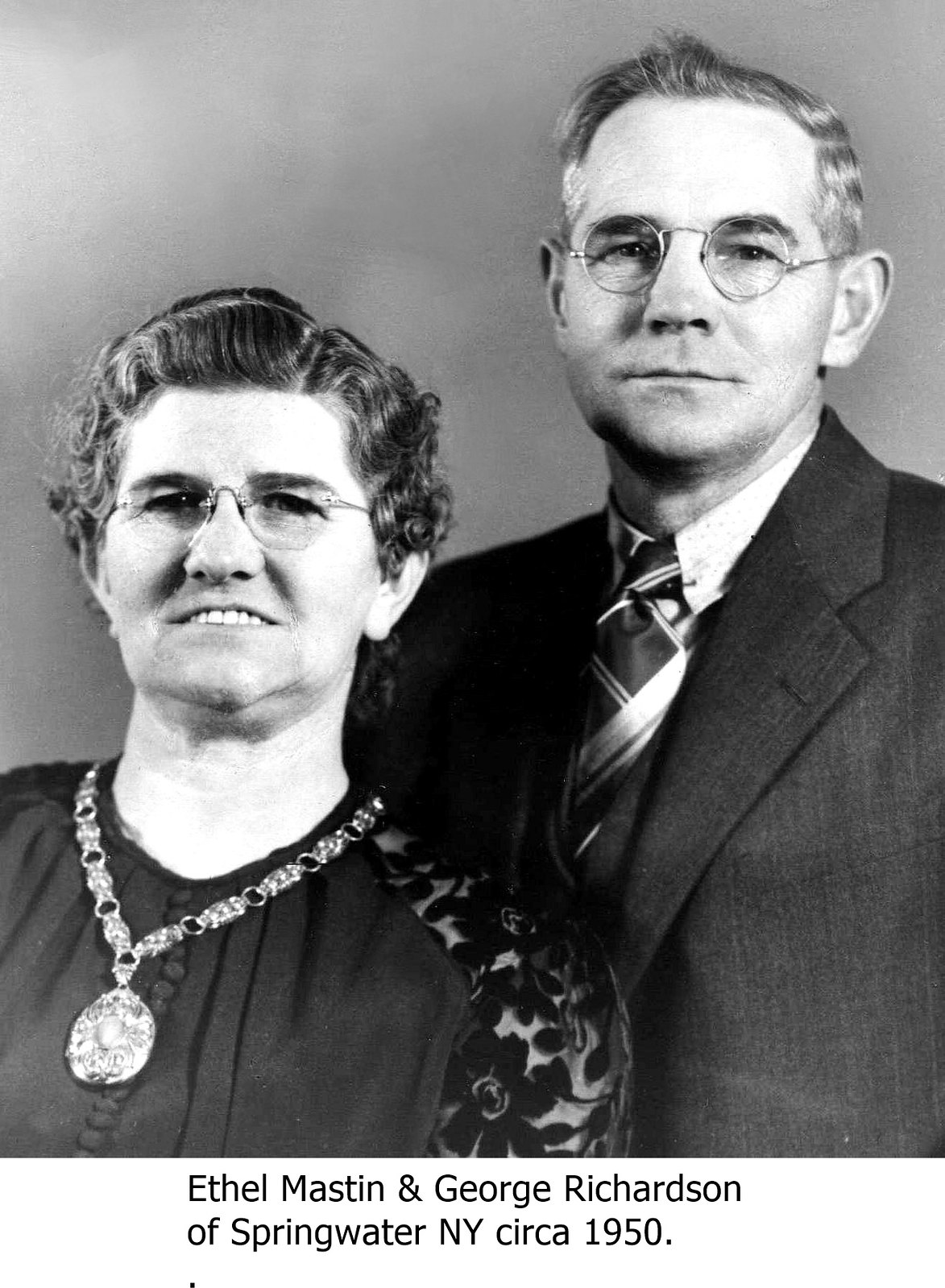The black-and-white photograph features Ethel Mastin and George Richardson of Springwater, New York, circa 1950, as stated by the caption beneath it. The couple is dressed formally, suggesting they are posing for a portrait. Ethel, standing on the left, has short curly hair, glasses, and a double chin, and is adorned with a large medallion necklace and a floral jacket. George, on the right, is taller and also wears glasses. He is dressed in a severe black suit with a striped tie, and his hair is short. Both are slightly smiling, with Ethel showing her teeth while George has more of a grin. The background of the photo appears gray and grainy, possibly suggesting a green screen or photo backdrop, which highlights the couple against a plain setting.